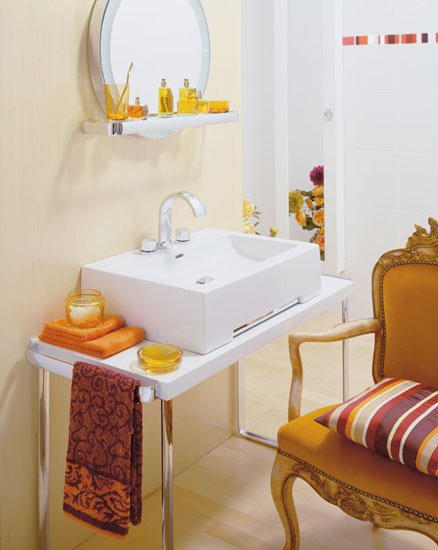The image depicts a brightly lit bathroom interior, centered around a pristine white porcelain sink with sleek silver faucets and knobs. Atop the sink rests a white tray, neatly organized with vibrant yellow cups and spray bottles. Above the sink, a large mirror framed in silver reflects the light, enhancing the room's brightness. 

To the left of the sink, a handle hosts a draped, patterned orange towel adorned with black, curvy spiral lines. Below the sink, a wooden table supports it, while a yellow dish and a matching yellow jar sit on the table's bottom right corner. On the bottom left, another orange towel adds a pop of color to the scene.

Adjacent to the table stands a chair with an orange cushioned seat and backrest, complemented by wooden armrests. The chair is dressed up with a striped pillow featuring alternating red, white, orange, and gray stripes.

The bathroom floor is elegantly laid with white wood tiles, accented by a subtle striped color pattern that runs along the base. In the background, an intricate floor arrangement adds a touch of sophistication to the room’s overall design.